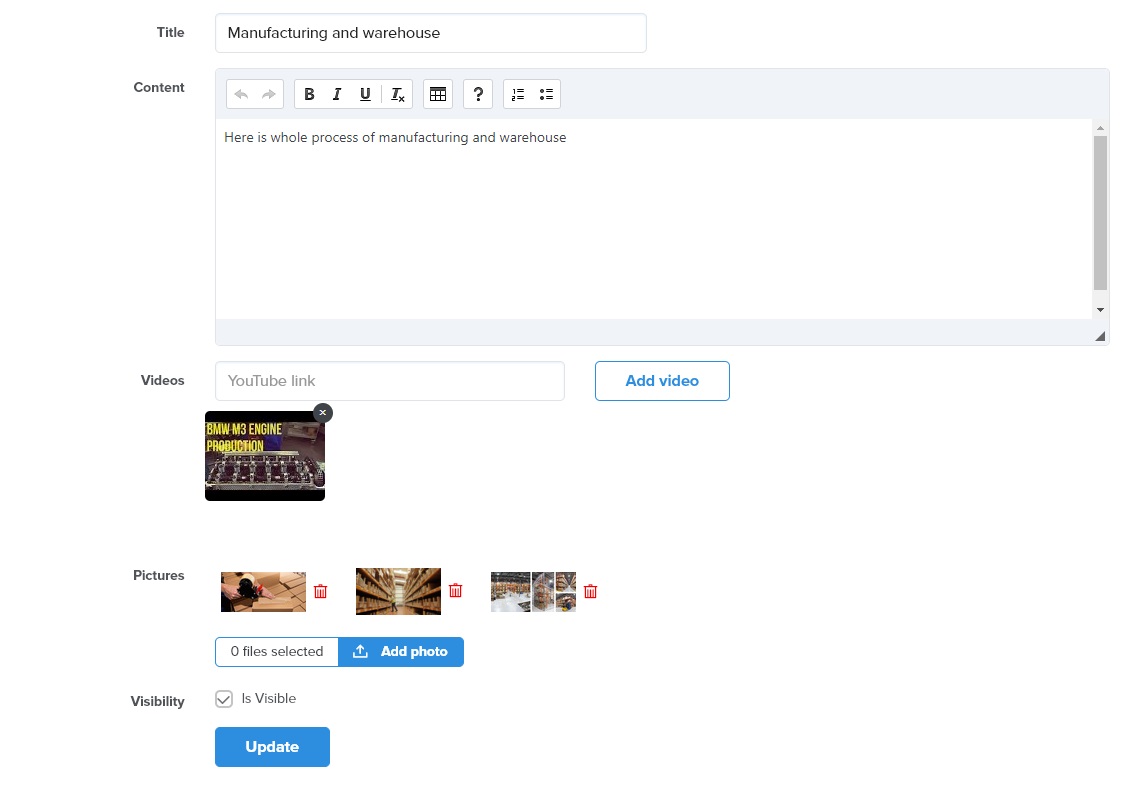The image appears to be a screenshot of a webpage or digital document template displayed on a computer screen. At the top of the screen, there is a horizontal navigation bar. On the left side, this bar includes the label “Title,” and displays the text “Manufacturing and Warehouse.”

Below this, there is a large rectangular text area labeled "Content" on the left. Inside this box, someone has typed, “Here is the whole process of manufacturing and warehouse.” Above this content box are various text formatting options.

To the far left of the content section, there is a vertical sidebar labeled "Videos," with a section to the right containing a URL text field and an “Add Video” button. Underneath this, there is a thumbnail image of a YouTube video titled "BMW M3 Engine Production."

Following the videos section is a "Pictures" section. This contains three images aligned horizontally, each accompanied by a red trash can icon to the right, presumably for deleting the images. Below this section, there is a file uploader labeled "0 files selected" alongside an “Add Photo” button.

At the bottom left of the screen, there is a "Visibility" section. This contains a checkbox labeled “Is Visible,” which is checked. Directly below this, there is a blue button labeled “Update.”